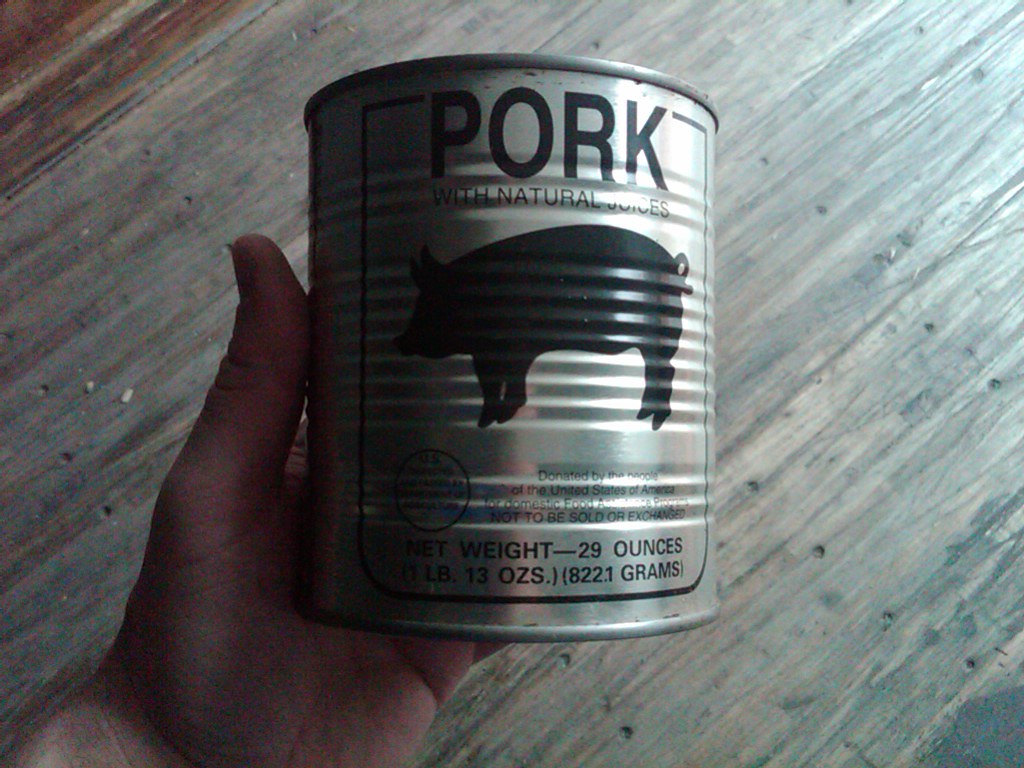This color photograph, though slightly low-resolution with noticeable pixelation, captures a left hand holding a metallic food can against a grayish wooden surface with black streaks—it might be a countertop, table, or floor. The hand, likely a white male's given the visible skin tone, is positioned with the thumb pointing upwards toward the top of the image. The can prominently displays the word "PORK" in large black letters at the top, followed by the smaller text "with natural juices" underneath, despite some overexposure. Below this text is a black silhouette of a pig, oriented with its head slightly downwards to the left, showing four trotters and a curly tail. Additional text on the can includes a message indicating it was "donated by the people of the United States of America for domestic food programs, not to be sold or exchanged," and it specifies the net weight as "29 ounces, 1 pound, 13 ounces, 822.1 grams." The bottom part of the can is slightly shadowed, obscuring some text, but emphasizing the weight details.